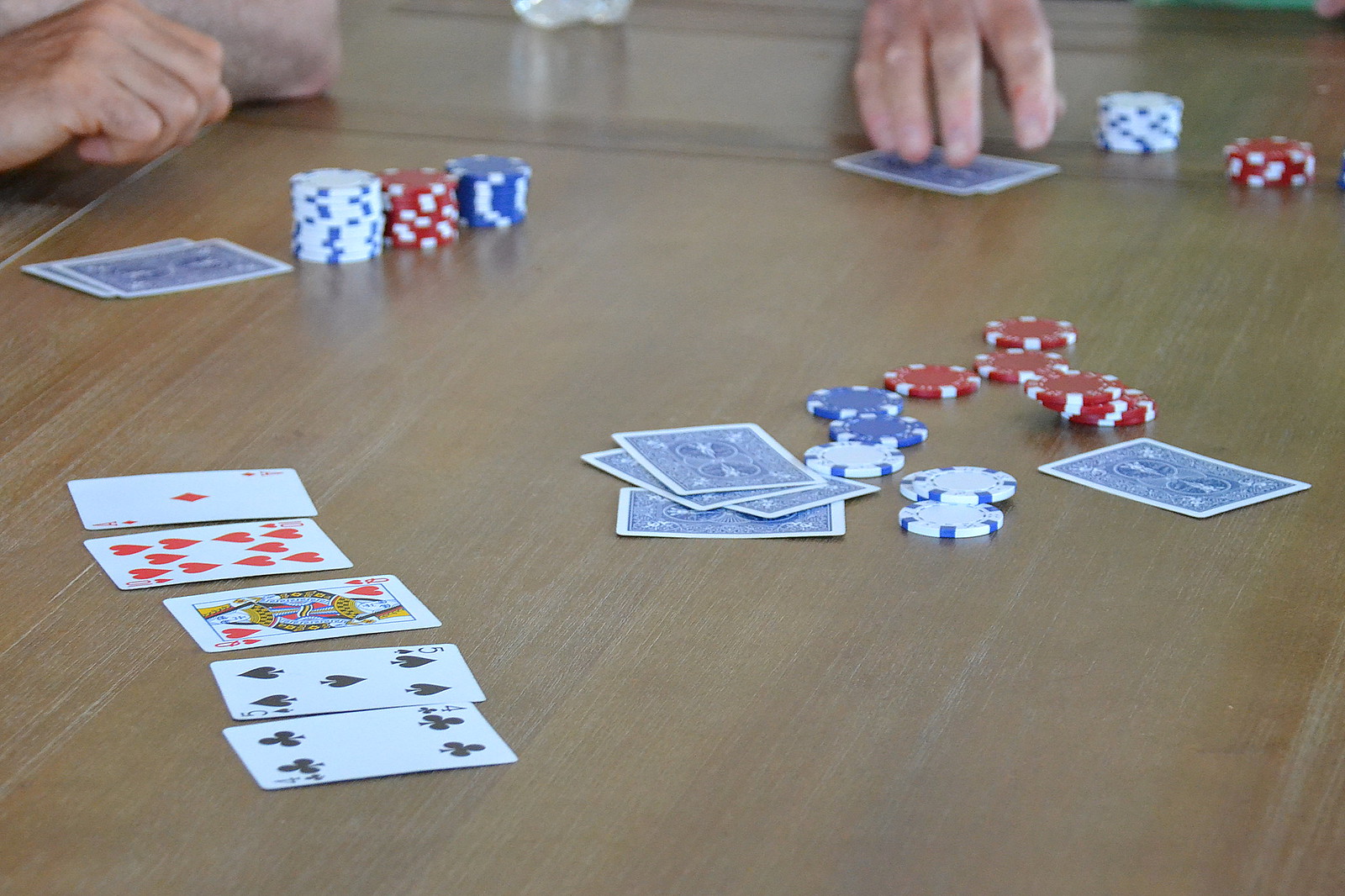On the table, a wooden light brown surface is visible, adorned with various items characteristic of a poker game. The bottom left corner features a spread of cards, including the Ace of Diamonds, Ten of Hearts, Queen of Hearts, Five of Spades, and Four of Clubs. Toward the top of the table, two players are faintly visible through their hands and poker chips. 

The player on the left has two cards face-down in front of them, with neatly stacked chips comprising white, red, and blue varieties, all approximately the same height. Conversely, the player on the right also has two face-down cards but possesses only a stack of white and a smaller stack of red chips.

In the center of the table, a small collection of muck cards lie face-down, flanked by a scatter of poker chips—six red, two blue, and three white. The card backs feature a distinctive blue design, while the poker chips display intricate patterns: red chips adorned with white squares on the edges, blue chips with white squares, and white chips with blue squares, adding a touch of elegance to the scene.